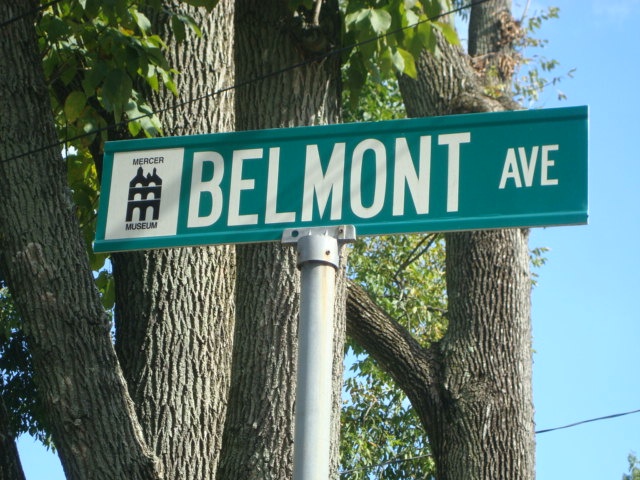In this bright and sunny photo, the main focus is on a green street sign that prominently displays "Belmont Ave" in large white letters. The sign is mounted on a textured, silver-colored steel pole. To the left of the street name, there is a noticeable sticker for the Mercer Museum, which features a small black icon of a building. The background captures a beautiful blue sky and several old trees with rough bark and green leaves. Three electrical wires are visible, two in the upper left corner and one in the lower right corner of the image, adding to the detailed urban scene.